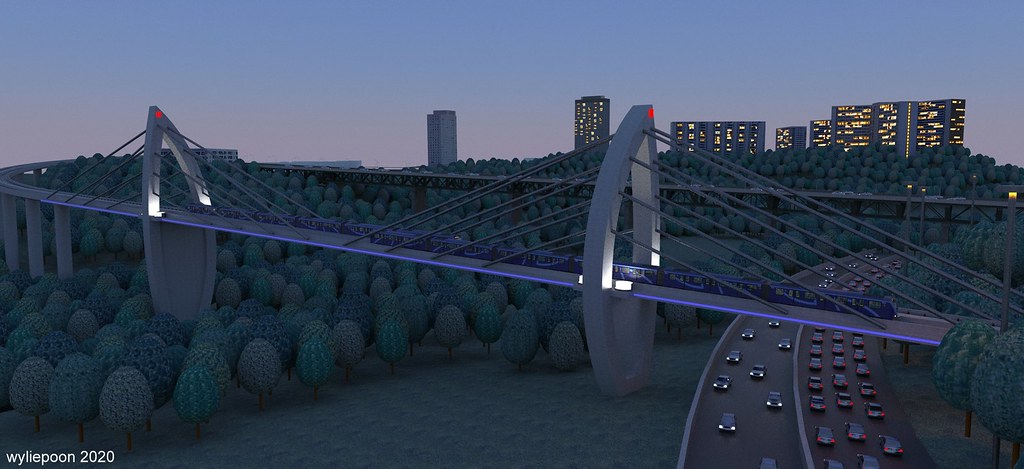This computer-generated rendering illustrates a futuristic bridge spanning across a busy highway set against the backdrop of a city at dusk. The bridge, gray in color and featuring a unique geometric design, arcs up to a point, creating an almost eye-shaped silhouette with curved sides. A sleek blue train glides along the bridge's span, which is supported by distinctive tear-shaped structures anchored to the ground and connected by an array of cables. The red circles at the top of these structures add a striking accent to the design. Beneath the bridge, the highway is seen with cars moving in both directions, their headlights cutting through the encroaching night. The scene is set in the evening, just after sunset, with the sky transitioning to a deep bluish-gray and a faint reddish hue illuminating the horizon. The city in the background, with its high-rise office buildings and skyscrapers, is aglow with yellow lights, while one solitary building remains unlit, standing apart from the others. A uniform forest of deciduous trees blankets the area under and around the highway, contributing to the overall symmetry of the scene. The image is signed "Wiley Poon 2020" in white letters in the bottom left corner.